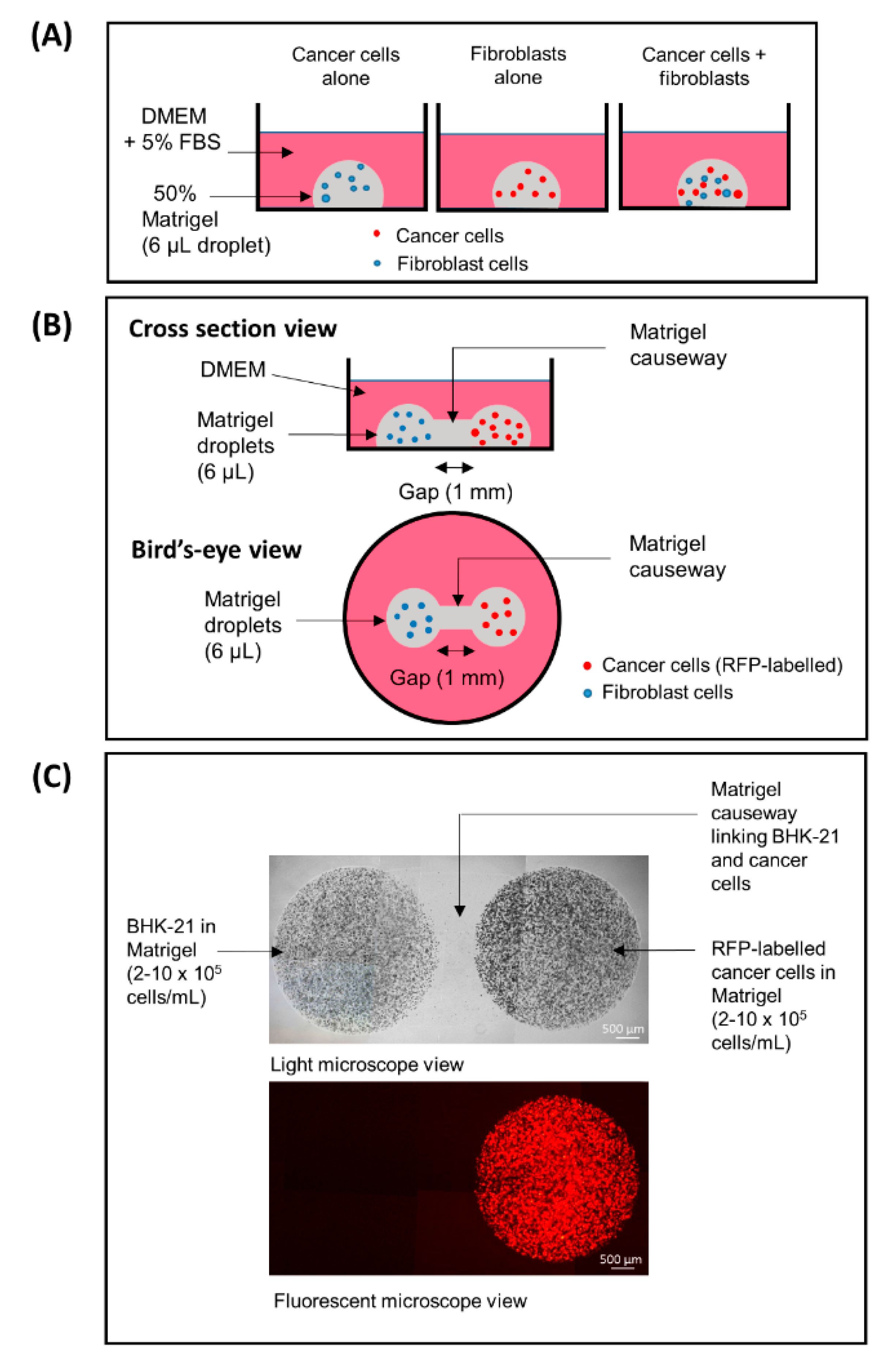This detailed medical diagram is divided into three sections labeled A, B, and C, arranged vertically. Section A, at the top, features three smaller diagrams illustrating different configurations of cancer cells and fibroblast cells using circular and semicircular shapes. The first diagram in A depicts cancer cells alone, represented by a gray semicircle at the bottom with blue dots inside, labeled "DMEM plus 5% FBS" and "50% matrigel 6UL droplet." The second diagram shows fibroblasts alone with red dots inside a similar gray semicircle. The third diagram illustrates a combination of cancer cells (red dots) and fibroblasts (blue dots) within the semicircle, labeled "cancer cells plus fibroblasts." Section B provides both a cross-section view and a bird's eye view of these cells. The cross-section view shows two semicircles connected by a matrigel causeway with a 1mm gap between them, one containing blue dots (fibroblasts) and the other containing red dots (cancer cells). The bird's eye view is a pink circle with two inner semicircles separated by a 1mm gap; the left side contains blue dots (fibroblasts), and the right side contains red dots (cancer cells). Section C includes real images of these cells, showing two circles with a matrigel causeway between them under a light microscope view and a fluorescent microscope view of cancer cells labeled RFP, with one image showing red cells and labeled "500 UM."